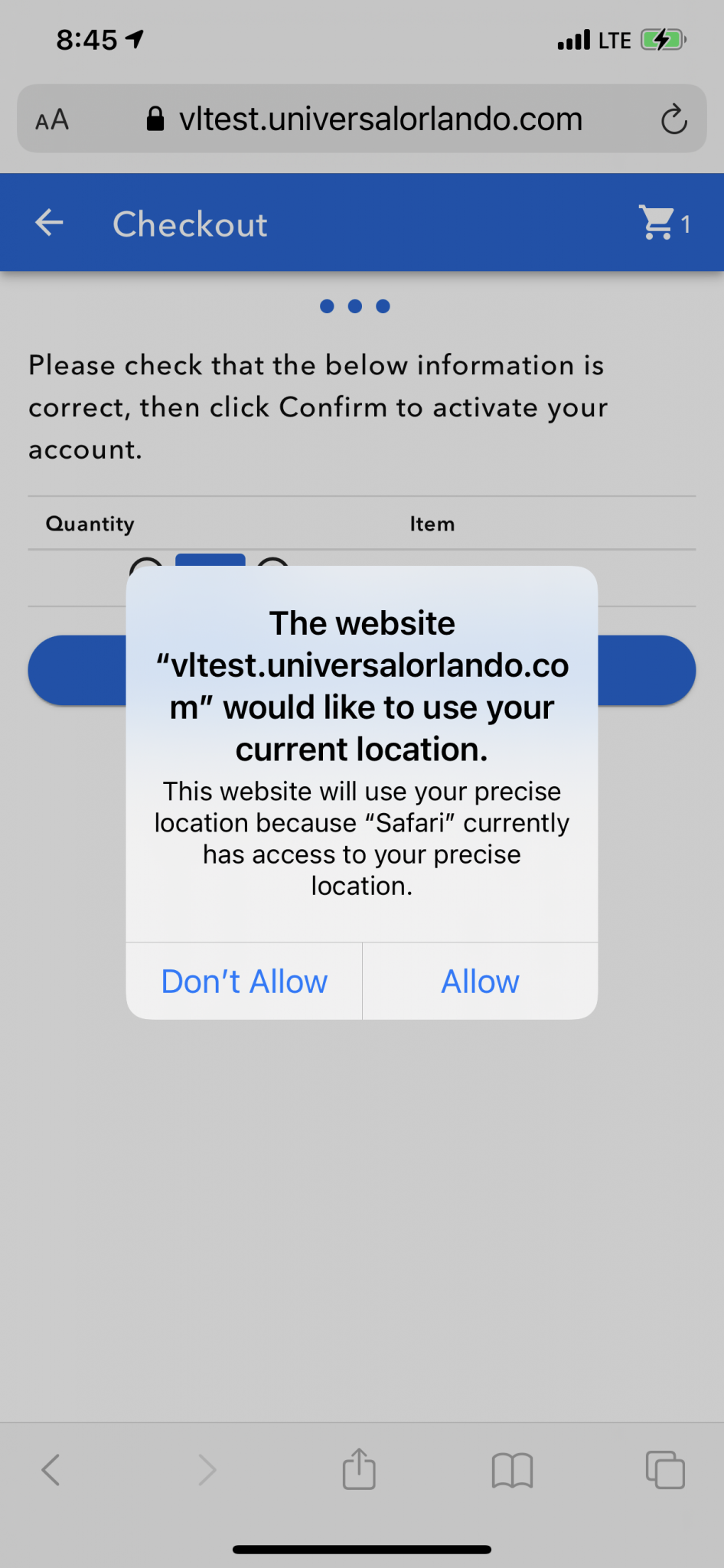A detailed screenshot of a smartphone display taken at 8:45 AM is shown. The phone is connected with full signal strength (4 bars) and has a fully charged battery. At the top of the screen, the Safari browser interface is visible, displaying the URL vltest.universalorlando.com, accompanied by a lock icon and two 'A's on the left side. On the far right, a refresh button is present.

Below the address bar, there is a prominent dark blue banner with a left-pointing arrow and the word "Checkout" next to it. A shopping cart icon is also displayed, indicating one item. Immediately beneath this banner, three blue circles are lined up horizontally.

Further down, in black text, the message reads: "Please check that the below information is correct, then click confirm to activate your account." Below this text, the words "Quantity" and "Item" can be seen. The rest of the information is obscured by a pop-up window.

The pop-up window prompts the user with information from the website, vltest.universalorlando.com, asking for permission to use the user’s current location. A message states, "This website will use your precise location because Safari currently has access to your precise location." There are two options at the bottom of the pop-up: "Allow" and "Don't Allow."